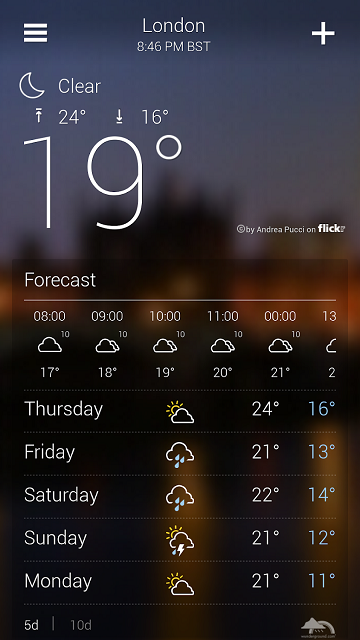This is a cell phone screenshot displaying the current weather conditions and forecast for London. The interface shows a mostly dark-themed blurred background of the night sky and a building. The top left corner features three horizontal lines, likely representing the menu icon. Centered at the top is the location "London," with the current time, "8:46 PM BST," displayed just below.

On the upper right-hand side, there's a prominent white plus sign, possibly for adding a new location or another feature. The weather icon is a moon, indicating nighttime with the "Clear" weather condition specified next to it. 

Current temperature details are prominently displayed: an upward arrow indicating a high of 24°C and a downward arrow signifying a low of 16°C. A large "19°" at the center represents the current temperature. Below this, the weather forecast for the upcoming days is listed, spanning from Thursday through Monday.